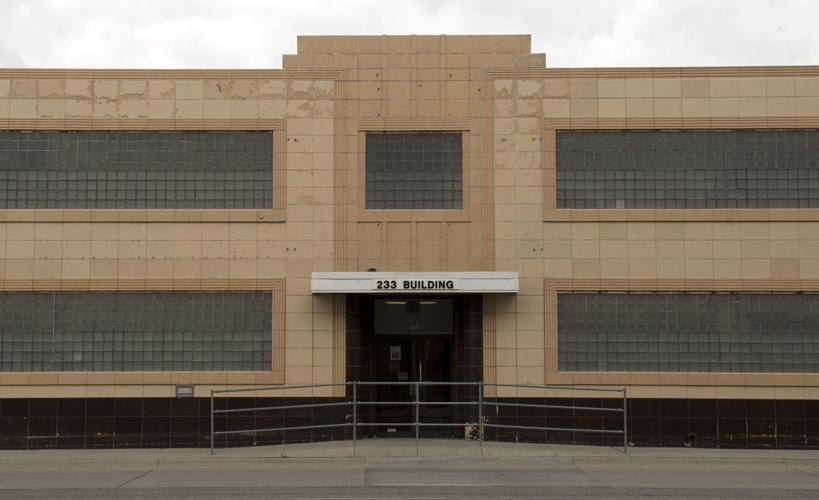This image depicts the exterior of a substantial, multi-story building that appears to be at least four stories high, though the presence of only two layers of windows suggests high ceilings within. The building is clad in tan stucco tiles with darker tan trim accentuating the windows and edges. It has a somewhat institutional, perhaps prison-like appearance, evoked by the barred windows arranged in long rectangular shapes, contributing to a rigid geometrical design. There are two such windows on either side of the entrance on each level, topped by a smaller, squarish window above the doors. The doors themselves are double glass doors set beneath a white awning that reads "233 Building" in black text. Flanking the entrance, there is a gray metal railing extending left and right, all set against a pale gray concrete sidewalk at the building's base. The sky overhead is filled with puffy clouds, adding a softer contrast to the building's stark facade.